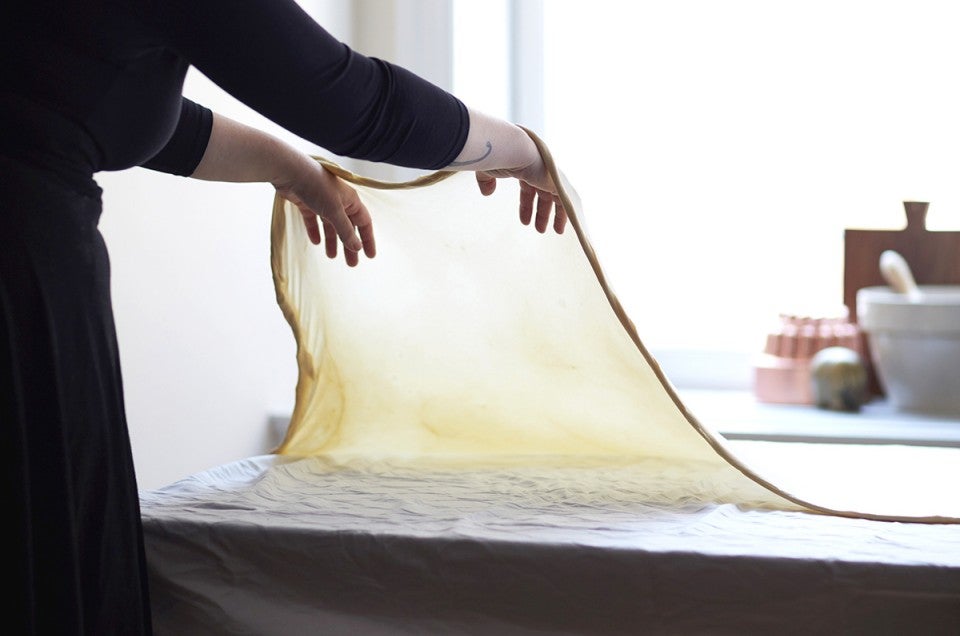This horizontal, full-color photograph, captures a Caucasian woman, seen from behind, engaged in a culinary activity in a well-lit room with natural light. The upper right corner of the image is bathed in whiteness, revealing a window frame in the upper center, hinting at an unseen outdoor scene. Dominating the left side of the image, the woman is dressed in a long black dress with sleeves rolled up to her mid-forearm, intensely focused on her task. She skillfully stretches an enormous, almost transparent dough, draped delicately over the backs of her hands, resembling thin fabric due to its extreme thinness and light cream-colored hue. The surface she works on appears to have a large white tablecloth. To her right, a mixing station features a large white bowl with a wooden handle protruding, a wooden cutting board, and a pink dish. The scene is a captivating blend of precise kitchen activity and the serene simplicity of natural light.